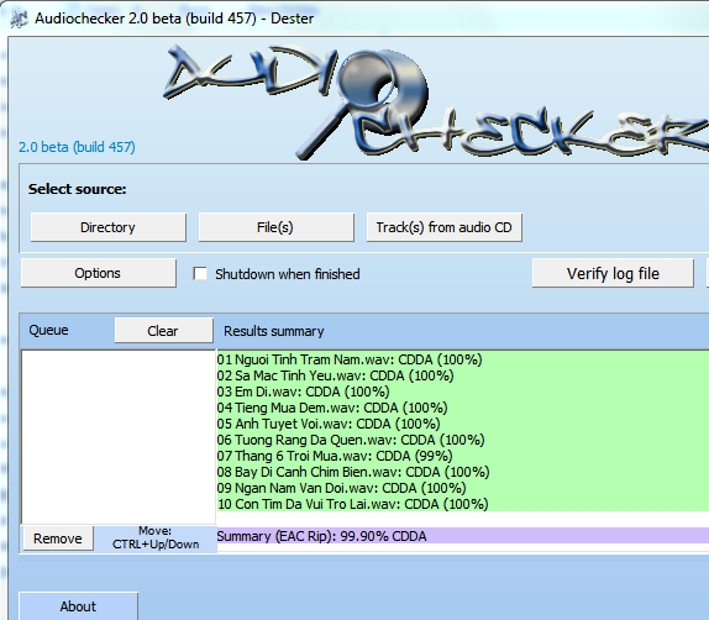The image is a screen grab of a Windows application called AudioChecker 2.0 Beta (Build 457 - Dester). The software interface is primarily light blue with elements of white scattered throughout the borders. The heading at the top of the screen features black text reading "AudioChecker 2.0 Beta (Build 457 - Dester)", accompanied by a unique logo where a graffiti-style "AudioChecker" font is used. A magnifying glass graphic notably zooms in on the letter "O" in "audio".

The interior of the user interface also has light blue backgrounds and presents blue text reiterating "AudioChecker 2.0 Beta (Build 457)". Below this, there is an indented section—still in light blue—that contains gray buttons with labels such as "Directory", "Files", "Tracks from Audio CD", "Verify Log", "File", "Options", and "Shutdown when finished". Additional options and actions include checkboxes, a queue system, and options to clear selected items.

Towards the bottom of the interface, a white rectangle appears next to a green rectangle with multiple lines of text. The green section displays results of the checks and operations performed by the software. The results section contains a list, with titles possibly in a Southeast Asian language, showing details and percentages such as "N-G-U-O-I-T-I-N-H-T-R-A-M-NAM.W-A-V-C-D-D-A 100%" and other CD-DA (Compact Disc Digital Audio) related information. Lastly, the interface includes a purple one-line section summarizing the program's actions, and at the very bottom, a button labeled "About".